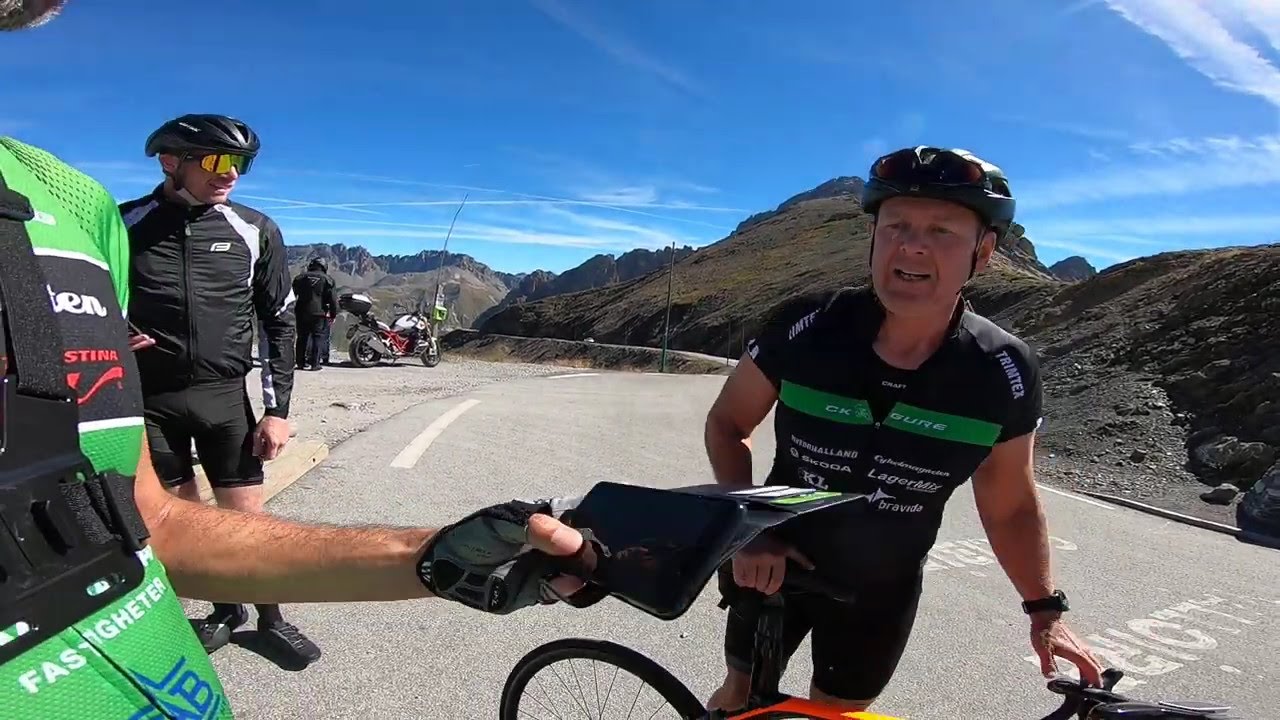The image captures a vivid scene of three men clad in coordinated biker gear, emphasizing green and black colors, indicative of their team or sponsors. At the forefront, one man, largely out of frame except for his chest and hand, extends a black wallet-like item filled with ID cards or credit cards towards a fellow biker. This man, who gazes down at the wallet, has his glasses and helmet lifted, revealing his intent stare. He’s gripping the handlebars of a red bike. The man holding out the wallet also seems to have an iPhone in his hand, its screen reflecting his face. Standing behind the man with the red bike, another individual, fully geared with his helmet and goggles on, looks on. In the background, more bikers can be spotted near a distant motorbike, suggesting the setting might be a marathon or bike race. The scene unfolds on a painted asphalt road stretching towards hills and rocky mountains, under a partly cloudy sky, encompassing a broad spectrum of colors like blue, gray, and brown, evoking the atmosphere of an outdoor, midday event.